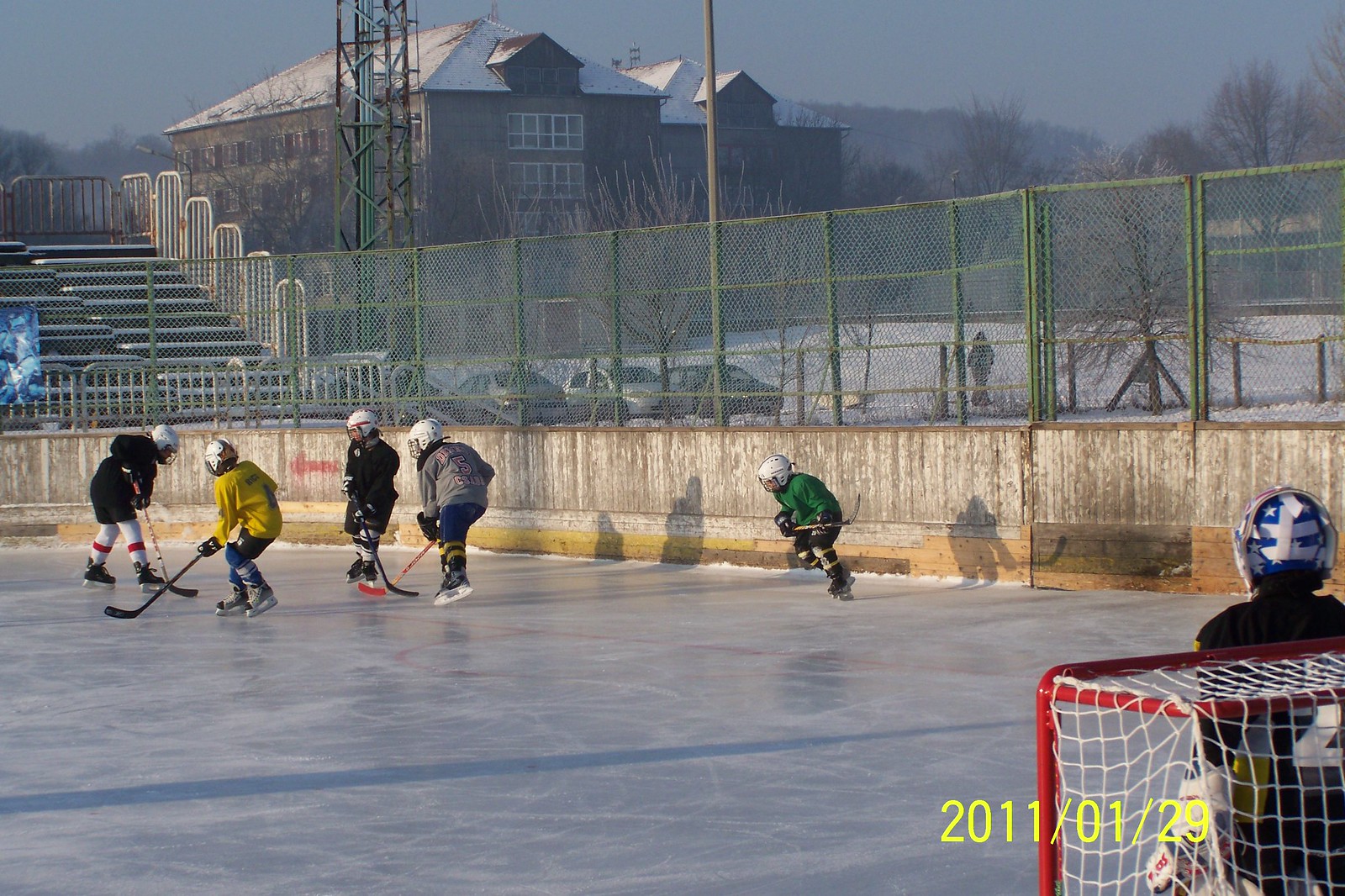The photo, dated January 29, 2011, captures an outdoor ice hockey game at a local skating rink surrounded by snow. In the foreground, a player donning a blue and white helmet with a white number two on his black jersey stands in front of a red-framed, white-netted goal positioned in the bottom right corner. The rink is encircled by a green chain-link fence and features empty bleachers covered in snow. The center-left area of the rink is alive with action as young players, dressed in various colored jerseys and white helmets, battle over the puck. The backdrop reveals a tall, four-to-five-story brick building with dormers, possibly a school or university, and an open metallic structure resembling an electrical or infrared cell tower. There are also parked cars and a snow-covered field behind the rink, adding to the wintry atmosphere. The date is prominently stamped at the bottom of the image in yellow letters: 2011/01/29.